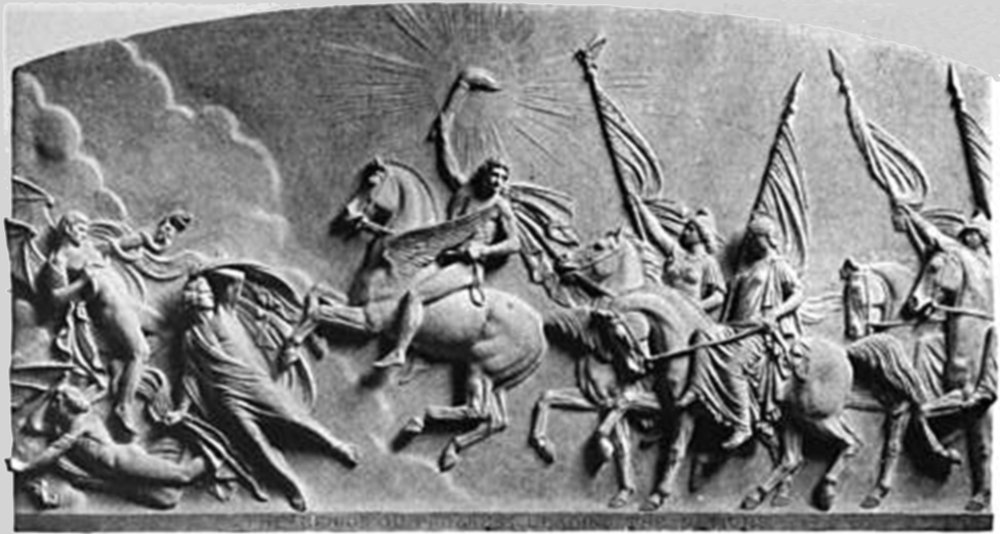The image depicts an intricate, detailed engraving or statue made from dark stone, reminiscent of ancient Greek or Roman art. The scene, carved in a half-circle shape with a rounded top and a flat bottom, portrays a tumultuous battle. Central to the composition are warriors on horseback, positioned primarily in the middle and to the right. These figures are armed with shields, spears adorned with flags, and one central figure holding a torch. They appear to be in the midst of driving out demonic figures, which are located in the bottom left corner. The overall coloration of the piece is monochromatic, featuring various shades of gray, slate, and white, lending a stark, solemn atmosphere to the depiction of conflict and struggle.